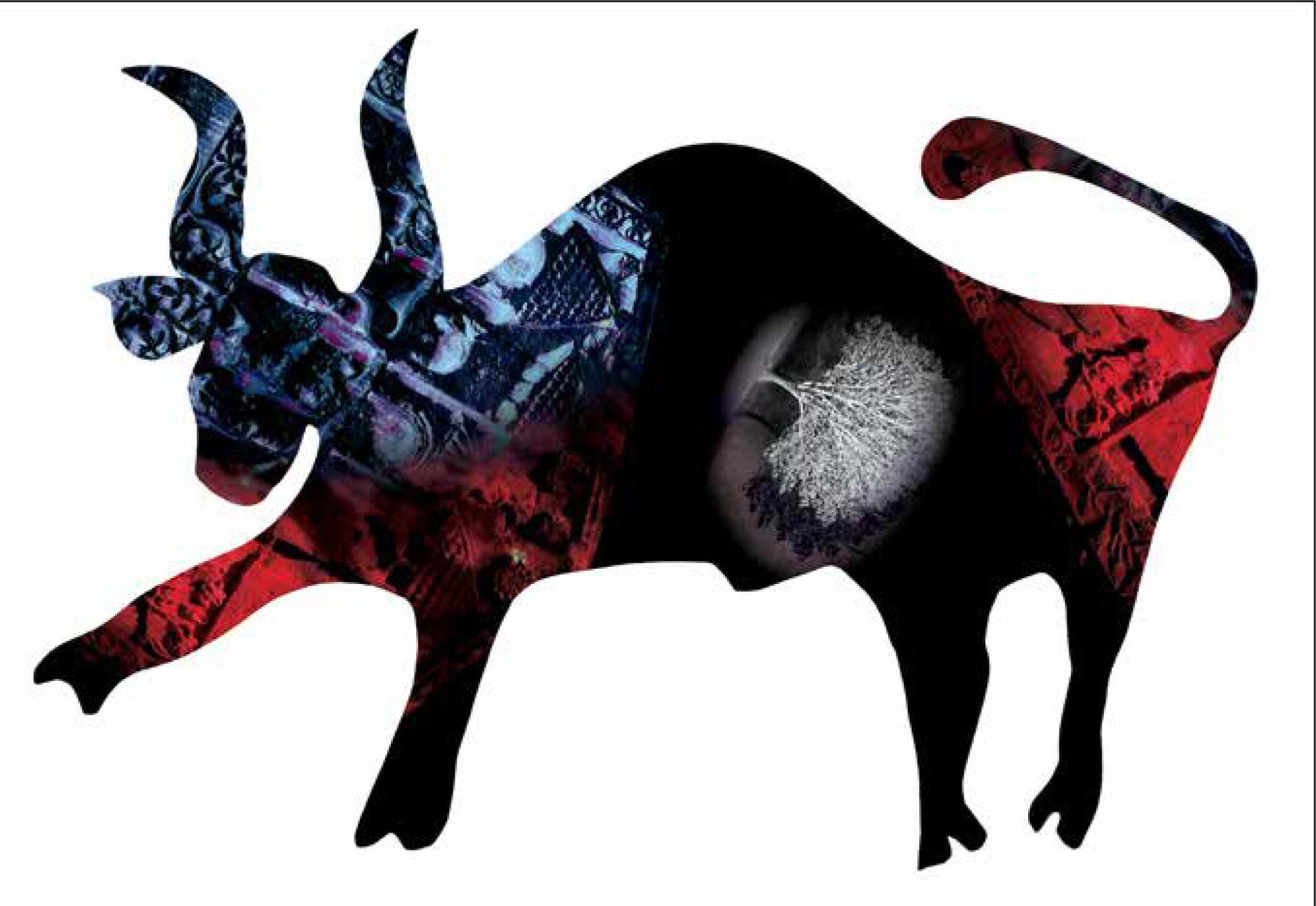The image features a horizontally aligned rectangular art piece with a black border along the top and the right side. The centerpiece is a detailed outline of a bull, filled with an intricate and colorful mixed media collage. The face and horns of the bull are adorned in black, blue, and purple hues with various intricate designs. The arms of the bull are bold in red and black, while its back is primarily black, displaying a striking hump. Notably, around the bull's stomach area, there is a circular cutout showcasing a black and white photograph of a tree tilted sideways, featuring a lonesome light source illuminating it and casting a shadow behind.

The collage inside the bull combines photorealistic images and artistic abstractions that resemble mechanical or circuitry-like designs, predominantly in blue, black, and red colors. The back legs are solid black, and the tail and rear end incorporate red and black with hints of blue and purple. All these elements come together on a plain white background, creating a visually compelling art piece that combines traditional drawing outlines with modern photographic and digital textures.